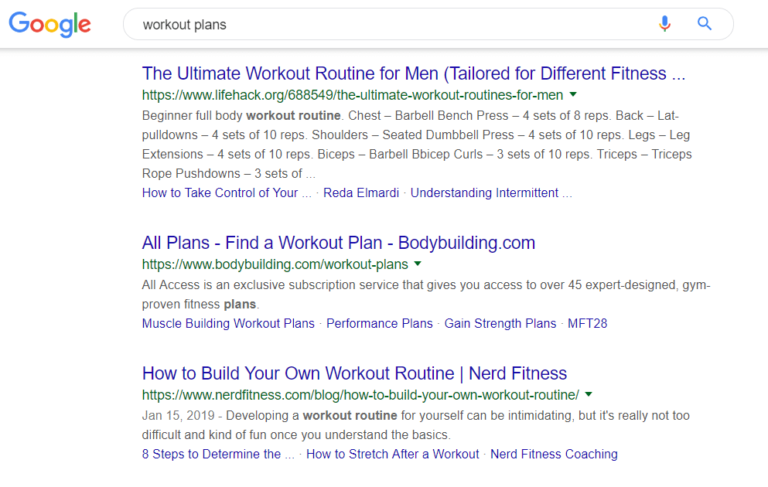Screenshot of a Google Search Results Page

At the top left corner of the web page, the iconic Google logo is displayed. Below it, a prominent rectangular search bar contains the text "workout plans," accompanied by a blue search button and a microphone icon located at the top right corner within the same row.

Three search results are returned on the page:

1. The first search result features the title "The Ultimate Workout Routine for Men" highlighted in blue, suggesting tailored plans for different fitness levels. Below the title, the website URL appears in green and provides a brief description of the content.

2. The second result is titled "All Plans: Find a Workout Plan from Bodybuilding.com," with the URL "bodybuilding.com/workoutplans" displayed underneath in green text. This result likely directs users to a comprehensive selection of workout plans available on Bodybuilding.com.

3. The third result is "How to Build Your Own Workout Routine" from Nerd Fitness. Its URL is listed in green as "www.nerdfitness.com/blog/how-to-build-your-own-workout-routine," offering a guide on creating custom workout routines.

The entire search results page is set against a clean, white background.